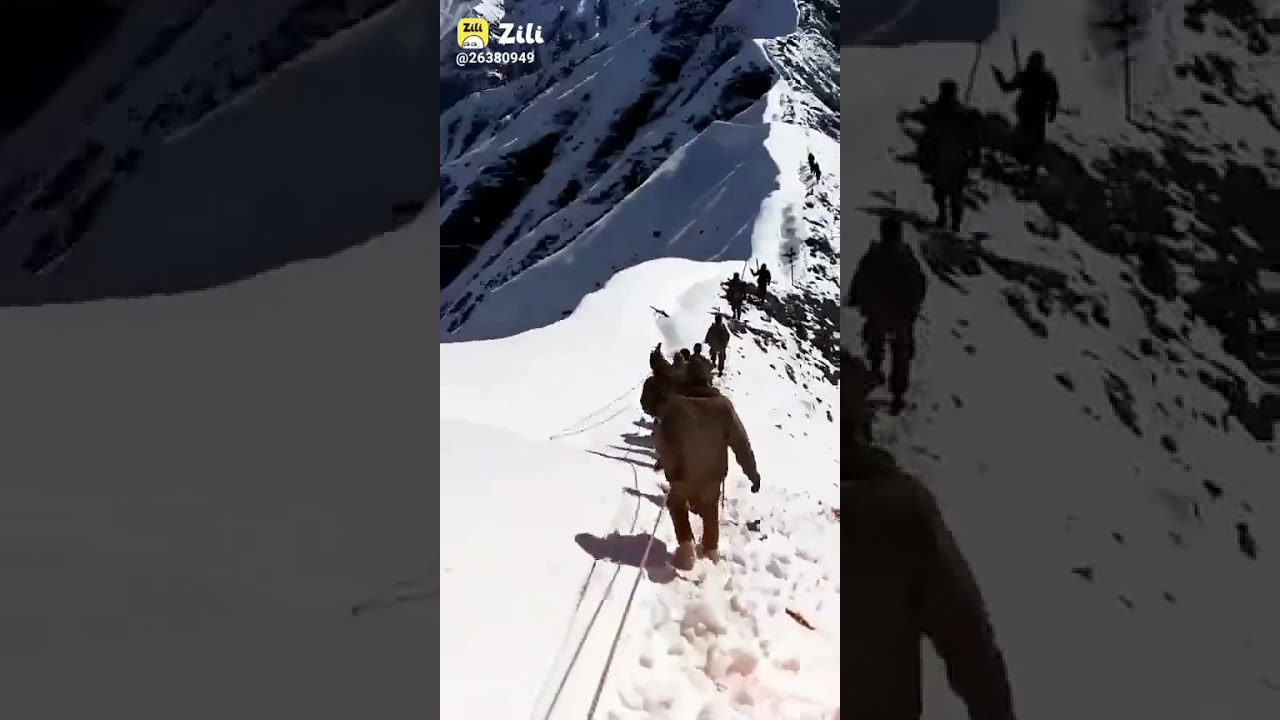This image captures a group of around a dozen people engaged in a challenging snow-covered mountain hike. Clad in thick winter clothing, brown and black jackets, snowshoes, and sturdy boots, they are navigating the treacherous ridge of a high mountain. The hikers are secured by a guide rope, aiding their descent across the rocky, snow-blanketed slopes. The scene, likely a screenshot from a vertical social media video, is bright and sunny, emphasizing the pristine, white expanse and rugged terrain. In the upper left corner of the image, the yellow Zilli logo features prominently, with "Z-I-L-I" in bold white font and the number sequence 263-80949 beneath it, indicating the video's source. The video appears to be framed with zoomed-in copies of the mountain scene on the sides, enhancing the central vertical view of the adventurers' path.